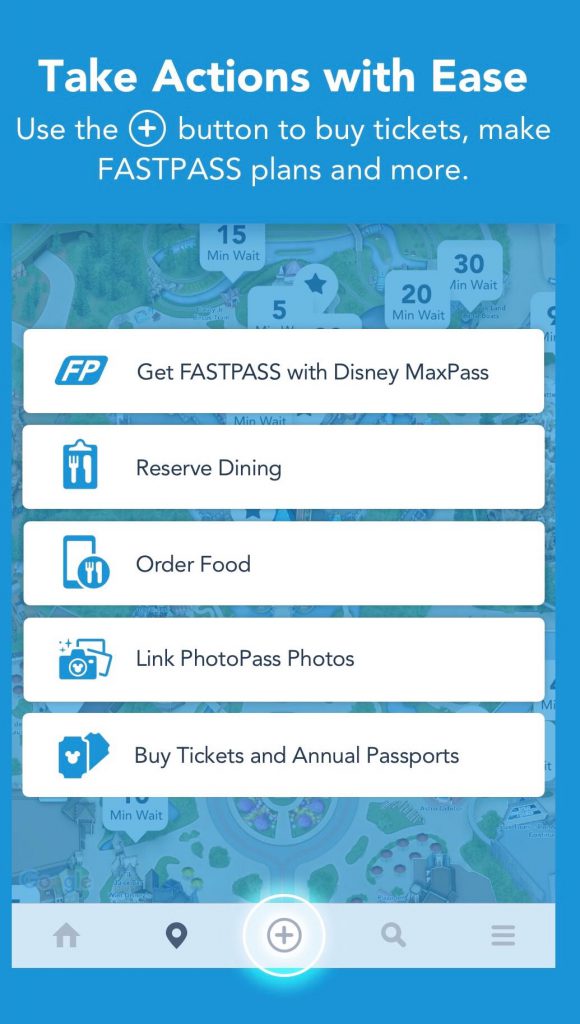Screenshot of an Android mobile app interface with a predominantly light blue background and white font detailing various features for user engagement. At the top, the text reads, "Take actions with ease. Use the plus button to buy tickets, make FASTPASS plans, and more." The "plus" button is encircled in white.

Behind this, a semi-transparent map is visible, showcasing wait times for various attractions highlighted within thought balloons, displaying 5, 15, 20, and 30-minute wait times. The map also features several locator icons marked with a navy blue star in their centers.

Below the map, there are several rectangular white action buttons:

1. **FP - Get FASTPASS with Disney MaxPass:** This button is accompanied by an "FP" logo.
2. **Reserve Dining:** Featuring a fork and spoon icon atop a clipboard logo.
3. **Order Food:** Displaying a mobile phone next to a spoon and fork.
4. **Link PhotoPass Photos:** Icon of a camera with photos behind it.
5. **Buy Tickets and Annual Passports:** Illustrated with ticket stubs.

In the foreground, there is a centrally placed "plus" button, flanked by several icons: 

- To the left: A black-bolded locator icon and a grayed-out house/home icon 
- To the right: A grayed-out magnifying glass and a settings icon (three stacked lines).

This detailed app screenshot showcases comprehensive navigational and functional elements designed for a seamless user experience.